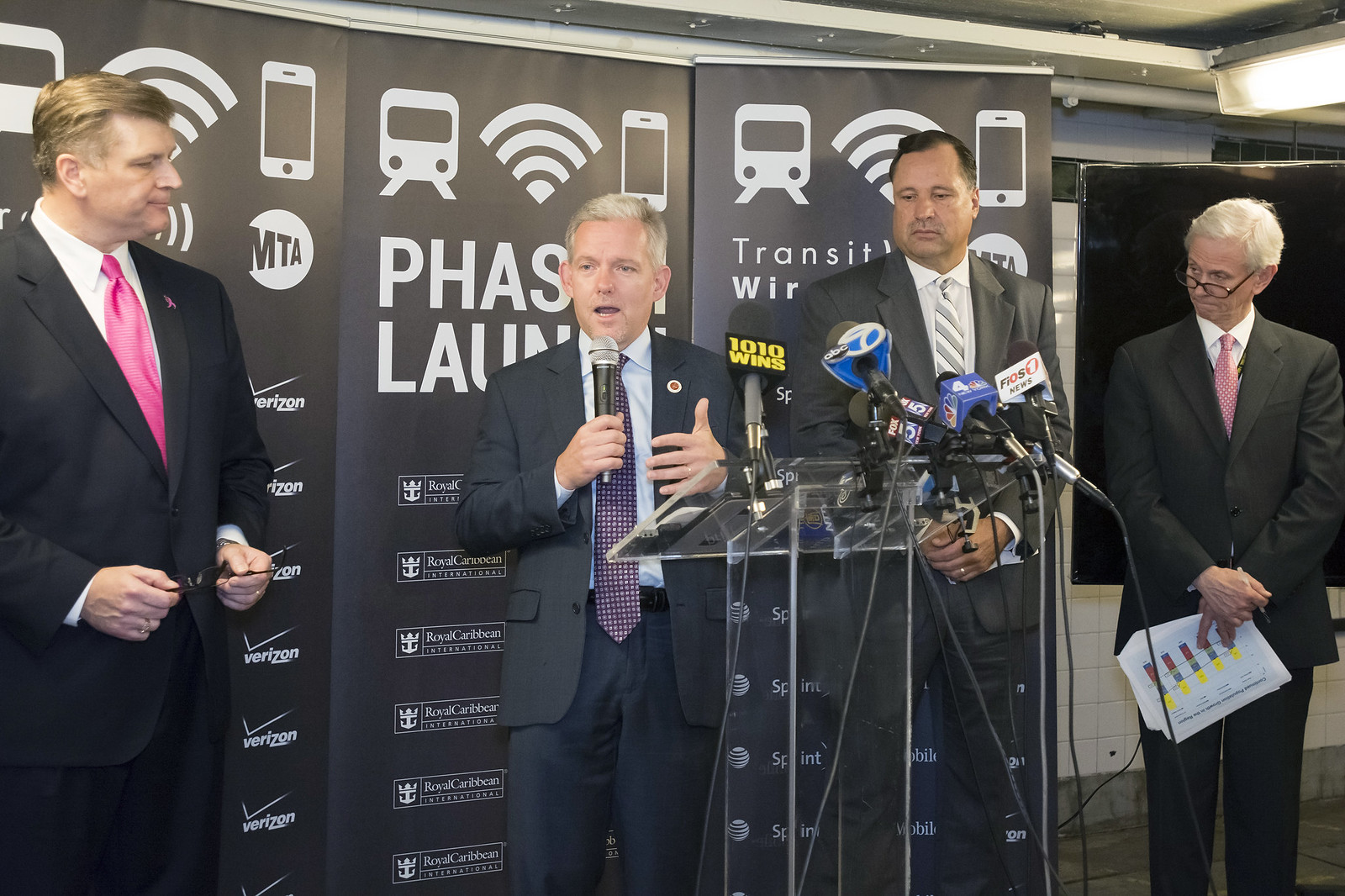In the image, a news conference is taking place with four gentlemen dressed in suits and ties, standing behind a transparent podium adorned with multiple microphones from media outlets such as NBC, Fox, ABC, Fios One News, and 1010 Wins. The central figure, a shorter man with gray hair wearing a dark blue suit and gesturing with his left hand, speaks into the microphone he holds in his right hand. To his left stands a taller man dressed in a dark blue suit with a pink tie, looking attentively at the speaker while holding his glasses. On the speaker's right, another man in a dark gray suit with dark hair stands with his hands crossed over the front of him. Furthest to the right is a smaller man in a black suit with dark-framed glasses, holding papers with bar graphs, indicative of discussing various statistics. The background features banners with symbols related to mass transit, including a cell phone signal icon and a smartphone image, suggesting they are discussing a new phase or launch related to wireless access in mass transit.